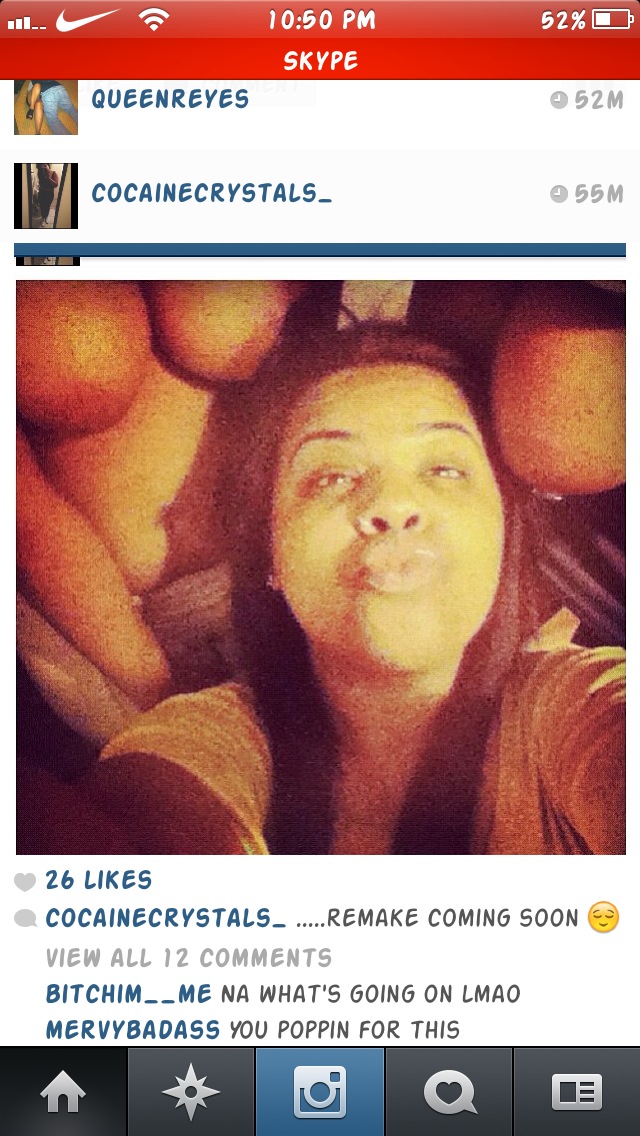A screenshot from a smartphone shows a young African American woman, likely in her 20s, taking a selfie for social media at 10:50 PM with 52% battery and displaying the Skype app at the top. She has long black hair, wears a white t-shirt, and strikes a duck face pose while facing the camera. Behind her, two women appear to be topless, their faces not visible, but their large breasts and bellies are discernible. The post, under the username "cocaine_crystals," has garnered 26 likes and reads "remake coming soon 😊." Comments from users include "nah, what's going on, LMAO" by BITCHIM__ME and "you poppin' for this" by MERVY_BADASS. The interface also displays typical smartphone elements such as signal bars, a Nike WiFi logo, and various icons for home, star, camera, heart, and messaging at the bottom.